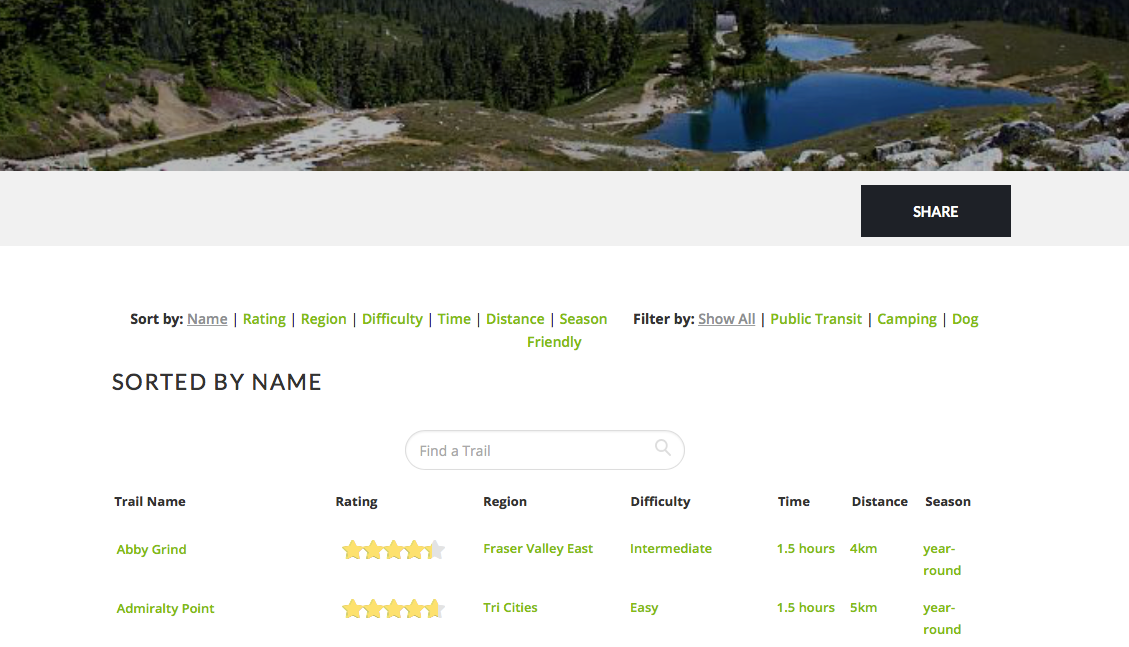The image showcases a detailed screenshot of a trail exploration app. The main portion of the image is a rectangular section displaying two adjacent bodies of water, each surrounded by lush, hilly greenery and scattered rocks, creating a picturesque trail landscape.

Beneath this scenic view is a gray bar featuring a black share button with white text. Below the share button is a white space, followed by an organized sorting and filtering interface. The sorting options, listed as "Sort by," include "Name," "Rating," "Region," "Difficulty," "Time," "Distance," and "Season Friendly," each separated by straight lines. The "Name" option is currently selected and underlined in gray, indicating alphabetical order from A to Z.

To the right of the sorting options is a "Filter by" section, with "Show All" in gray and underlined, indicating that all trails are being displayed. Additional filter options such as “Public Transit,” “Camping,” and “Dog-friendly” are listed in green text.

Further down, the screen displays a "Find a Trail" search bar and a search button for typing in queries. The trail information is organized into seven columns: "Trail Name," "Rating," "Region," "Difficulty," "Time," "Distance," and "Season." 

Two specific trails are highlighted: 
1. "Abbey Grind" – Rated 4.25 stars out of 5, located in Fraser Valley East, with an intermediate difficulty level. The trail takes 1.5 hours to complete, covers 4.4 kilometers, and is accessible year-round.
2. "Admiralty Point" – Rated 4.75 stars, located in Tri-Cities, with an easy difficulty level. This trail also takes 1.5 hours to complete, spans 5 kilometers, and is available year-round.